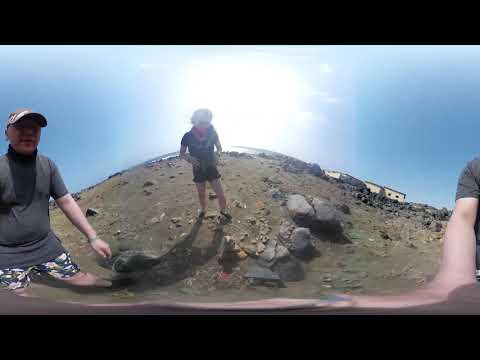In this heavily distorted 360-degree photograph, we see two individuals standing in an outdoor area that appears to be a beach, but the curvature of the lens creates an apparent hill in the landscape. The central figure is an older Caucasian male on the left, wearing a long gray shirt, floral swim trunks, and a light-colored baseball cap that casts a shadow over his face. His distorted right arm stretches along the bottom edge of the image, making it appear blurred and elongated. On the right side of the image, his left shoulder and arm are also visible due to the 360-degree effect. Another person, a woman, stands in the middle, dressed in black shorts and a dark gray shirt with a red scarf. She is looking down, standing on a rocky, stone-covered ground with various gray rocks and boulders scattered around. The ground is a light tannish-brown color. In the background, on the right, there are cream-colored buildings under a bright blue sky, with the sun shining brightly, adding to the distorted yet vivid quality of the photograph.